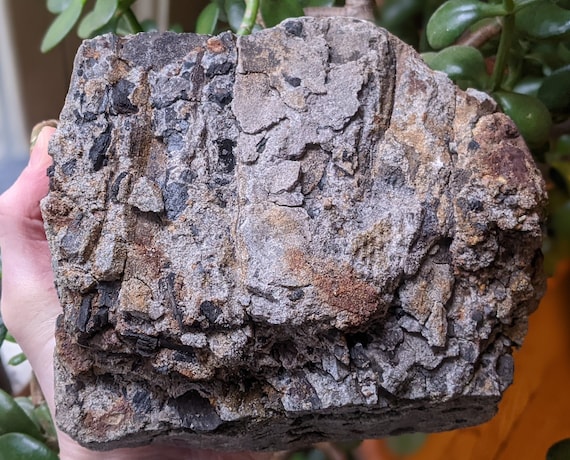The image features a hand prominently holding a large, jagged rock that dominates about 85% of the frame. The rock is rectangular with a curved top and exhibits a variety of muted colors, including shades of gray, brown, black, copper, and yellow. It has a notably flat base, suggesting it might serve as a display piece, suitable for a garden or tabletop setting. The background is clearly visible, revealing green leaves from a tree or plant and an orange object, possibly a bowl or wall, adding a subtle burst of color. The setting appears indoors, with a visible white wall or door in the upper left corner. The hand, mainly showcasing the thumb, firmly grasps the rock, making the mineral the central focus of the photograph.